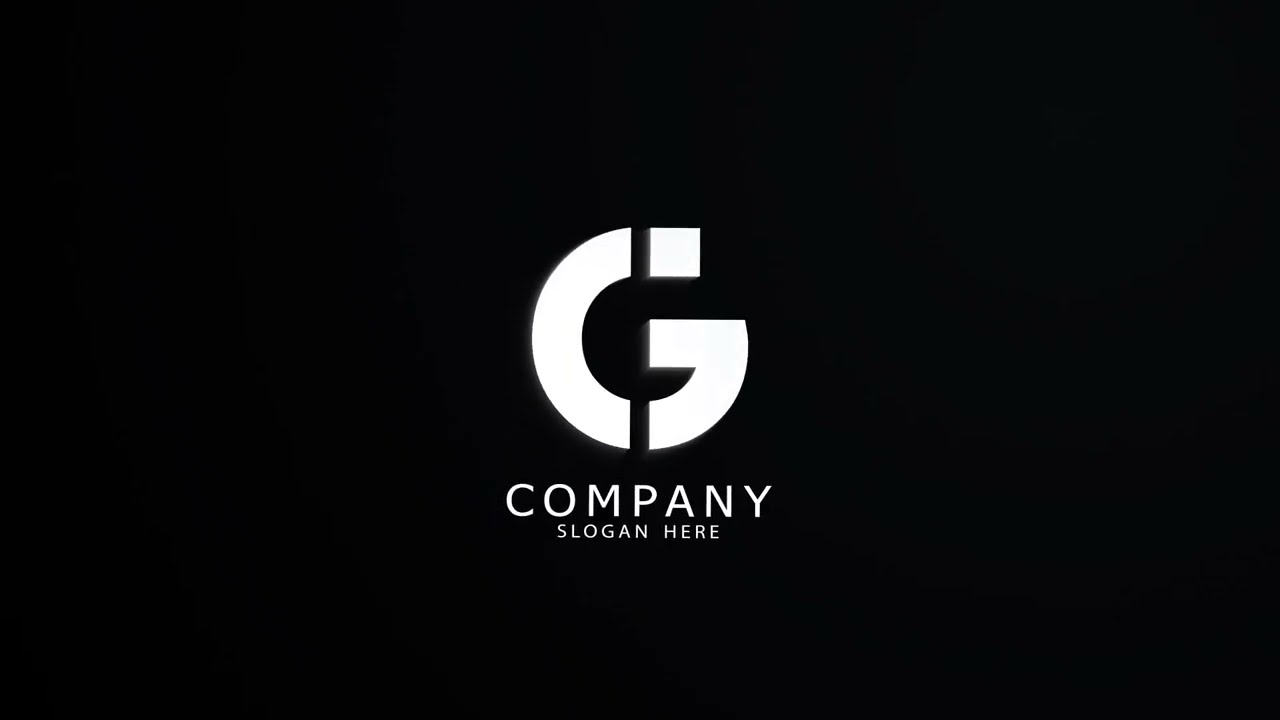The image is a horizontal rectangle, roughly one and a half times as wide as it is tall, with a stark, jet-black background. Centered in the middle of this black expanse is a prominent white letter "G," which is bisected vertically by a black line, giving it a split appearance. Directly below the "G," in larger white capital letters, is the word "COMPANY." Beneath that, in smaller white capital letters, is the placeholder text "SLOGAN HERE." Both lines of text are center-aligned. The overall design appears to be a rough draft of a company logo and slogan.